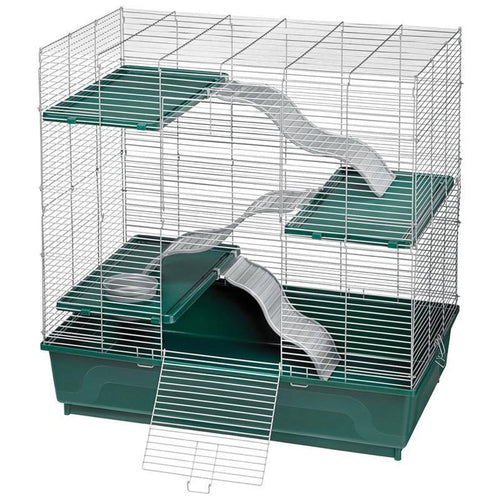This image displays a tall, multi-level rodent or bird cage set against a blank white background. The cage features a dark green plastic base that resembles a cat's litter box. Rising above it, the cage itself is composed of thin white metal bars. Inside, it has three green plastic shelves arranged in a staggered fashion: the first shelf is on the left, the second on the right, and the third shelf returns to the left at the top. Connecting these shelves are three wavy, silver-gray plastic ramps, creating a stair-like pathway throughout the cage. The cage's small square door at the bottom front is open and hinged downward. Additionally, there is a round silver dish situated on the first green shelf, which could serve as either a water or a food dish.